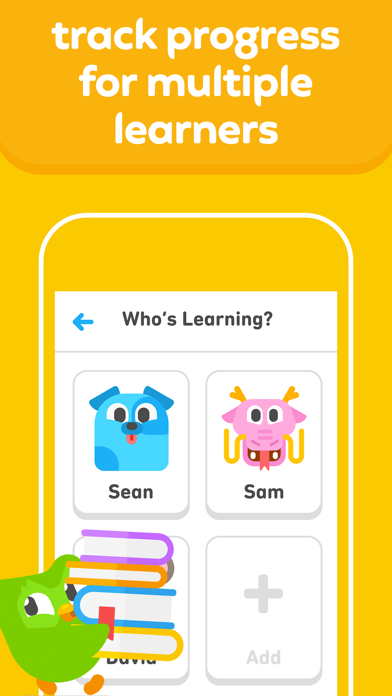In this image, the top portion of the background features an orange gradient that transitions into a slightly yellow but predominantly orange hue towards the bottom. At the top of the image, there's a header text in white that states, "Track progress for multiple learners." Below this, situated against the yellow background, is a square box. Inside this box is a detailed illustration of a frog positioned at the bottom left. The frog is green with black and white eyes and orange legs, and it is carrying a stack of books in purple, orange, blue, and yellow colors.

In the center of the white page, there's a black text that reads, "Who's learning?" To the left of this text is a blue arrow pointing right, indicative of navigation or a pointer.

Below this section, there are icons representing various learners. The first learner icon is of a blue dog, signifying one individual. On the top right, another learner is represented by an icon of a pink dragon with yellow horns, white teeth, and red lips; the learner's name is "Sam." On the bottom left, another learner's icon and name are partially obscured by the frog and its stack of books, making it hidden from view.

Finally, at the bottom right of the image, there's a space designated for adding another learner, marked by a plus sign and the text "Add."